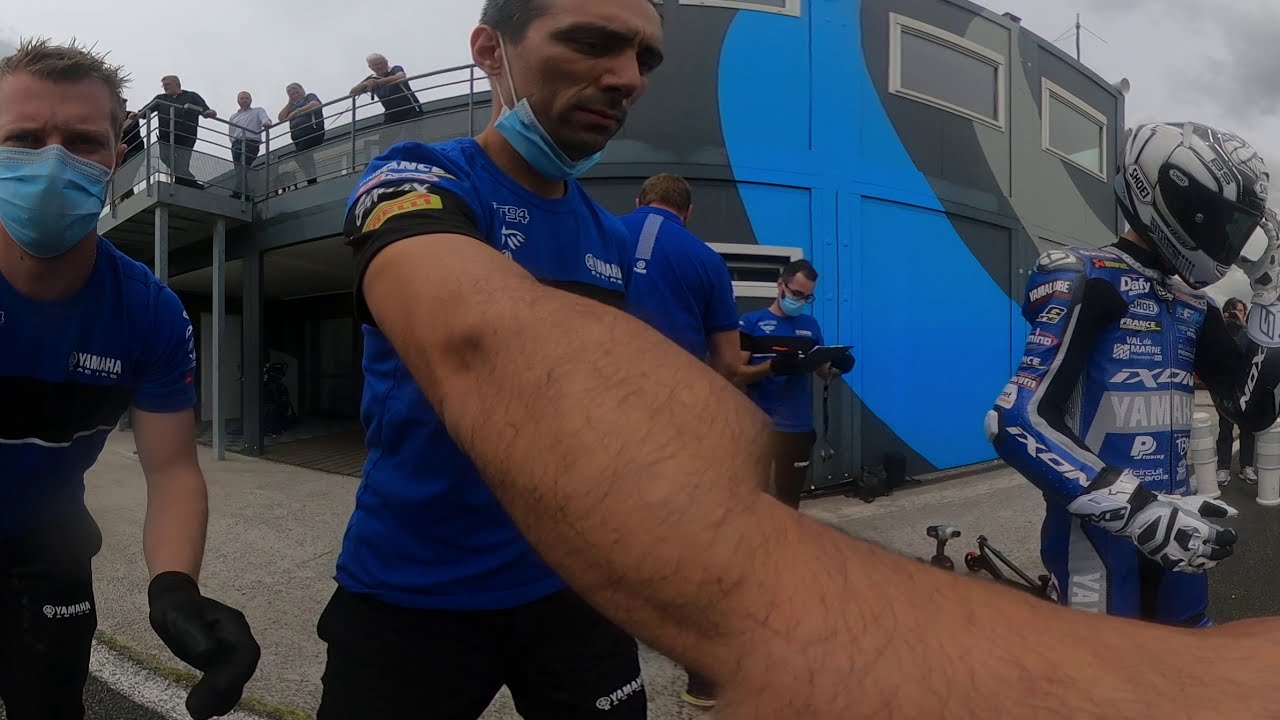The photograph captures a motocross racing scene featuring a group of individuals, primarily dressed in coordinated blue and black uniforms with various advertisements. Dominating the right side is a race car driver, identifiable by his full-body suit decorated with sponsorship logos such as Yamaha, Exxon, and others, along with a matching helmet that obscures his face. His suit is predominantly blue, gray, and black, complemented by gray and black gloves. 

To the left of him are several team members, some of whom are wearing blue face masks and black gloves, indicative of a COVID-19 precaution. They appear concerned, possibly tending to someone injured. The team members are clad in blue shirts and black pants, each bearing the Yamaha logo in white. One is holding a clipboard, and another a tablet, suggesting they might be engaged in some logistical support or recording of data.

In the background, a curved building with blue and gray stripes can be seen. Atop this structure, a spectator area with railings is visible, occupied by several onlookers dressed predominantly in dark clothing, with one person in a white shirt standing out. The sky above is overcast, dark, and threatening rain, reinforcing a dramatic atmosphere typical of a high-stakes racing event.